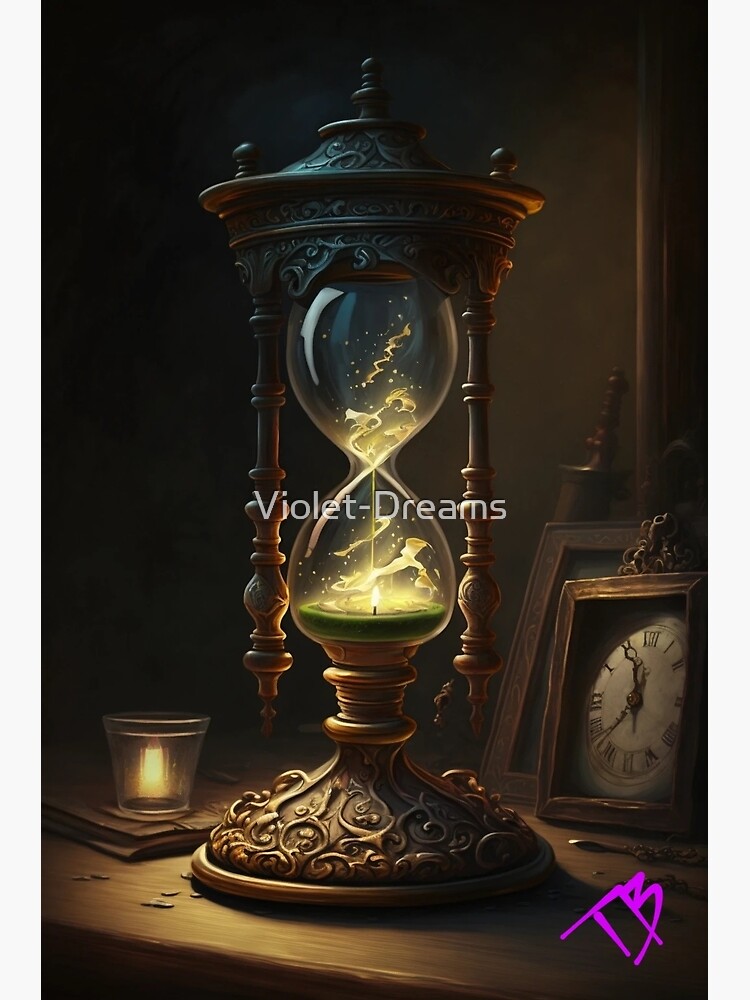The image titled "Violet Dreams" prominently features a highly detailed, 3D realistic hourglass with a wooden frame and clear glass, positioned on a wooden surface that might be a nightstand or end table. The hourglass does not contain traditional sand but rather a mesmerizing, magical yellow liquid spinning inside. Adding to its enchanting ambiance, a candle, possibly white and in a jar, is placed on the table, possibly atop a book.

On the right side of the image, a wooden-framed clock with Roman numerals is visible, featuring a white face with black hands and numerals against a brown wall. The background is complemented by a warm atmosphere due to the wooden elements and subtle lighting.

The entire scene is overlaid with a copyright transparent text that says "Violet Dreams" in white letters, and the bottom right corner bears the initials "TB" in purple, suggesting the creator’s signature, photoshopped onto the image. The visual composition and detailed elements create a visually captivating and unique artwork, blending realism with a touch of fantasy.